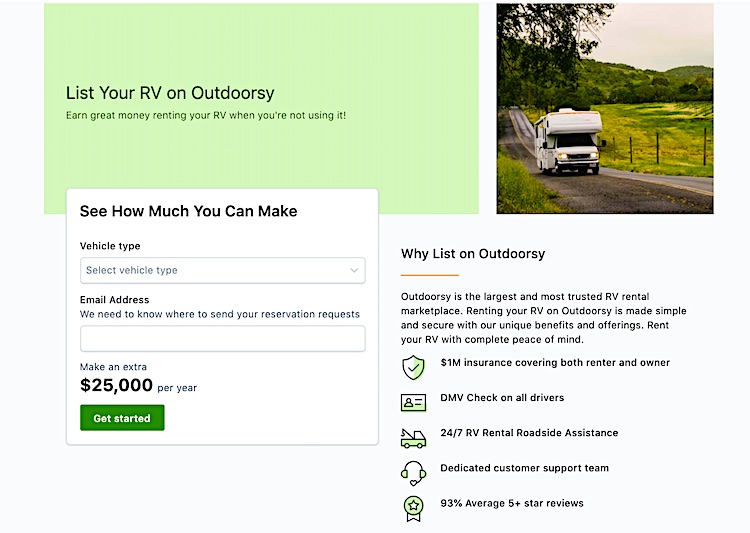The image depicts a webpage from the RV rental website Outdoorsy. Dominating the right-hand side, there is a picturesque photograph of an RV traveling down a rural road. The RV is situated adjacent to a gravel area beside a countryside road, featuring rolling hills and a wire fence supported by metal posts. On the left-hand side, a prominent green square displays the text "List your RV on Outdoorsy." Just below, in the same green square, the text reads, "Earn great money renting your RV when you're not using it." Under this section, a white block is visible, labeled "See how much you can make." This block includes a drop-down selection box labeled "Select vehicle type," followed by a text input box labeled "Email address." At the bottom of the white block, a green button invites users to "Get Started."